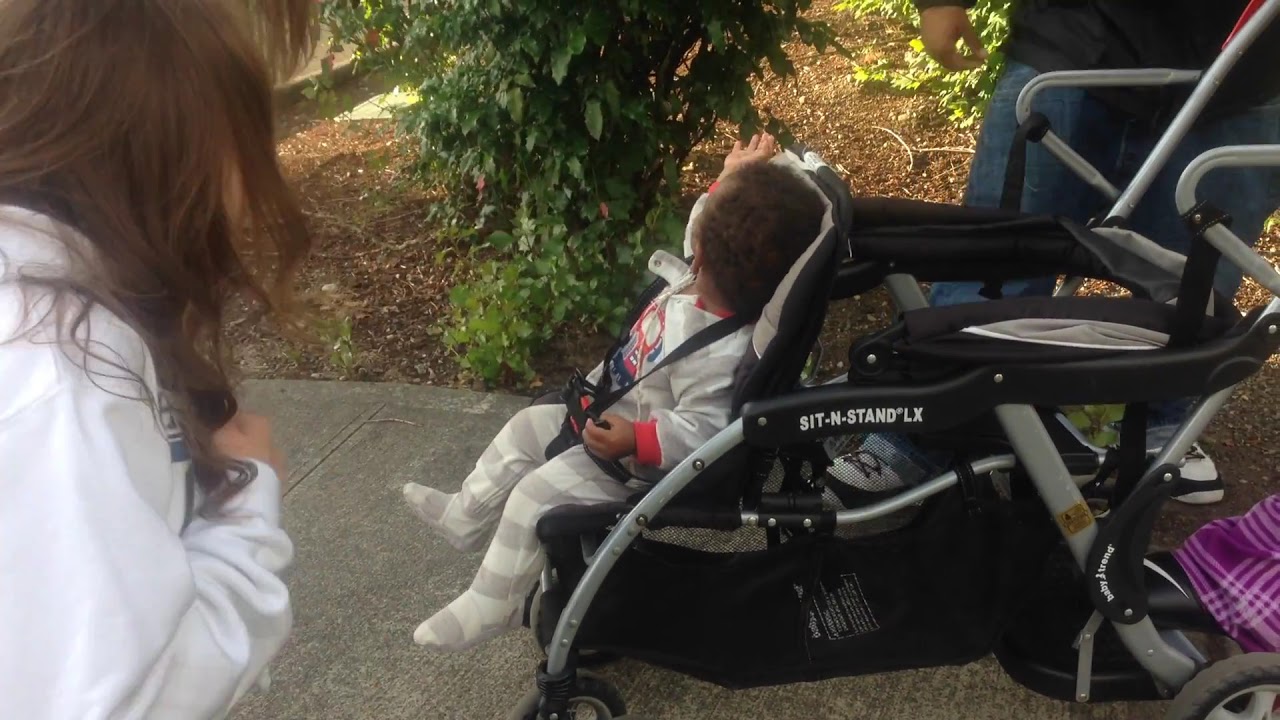In the image, a small child, wearing a gray and white striped onesie adorned with a red and blue vehicle, sits in a black and gray baby stroller marked with the white text "Sit and Stand LX" on the side. The child is looking upwards, seemingly captivated by something above. To the left of the stroller stands a woman with long brunette hair, dressed in a white hoodie with blue lettering, her attention directed towards the baby. Her face is partially obscured as she looks down at the child. Behind the stroller, a man is visible from the waist down, clad in blue jeans, white and black shoes, and a dark gray jacket. The scene is set on a dark gray cement sidewalk, surrounded by a hint of greenery, with a tree and some grass visible in the background, suggesting a casual outdoor moment captured in the photograph.